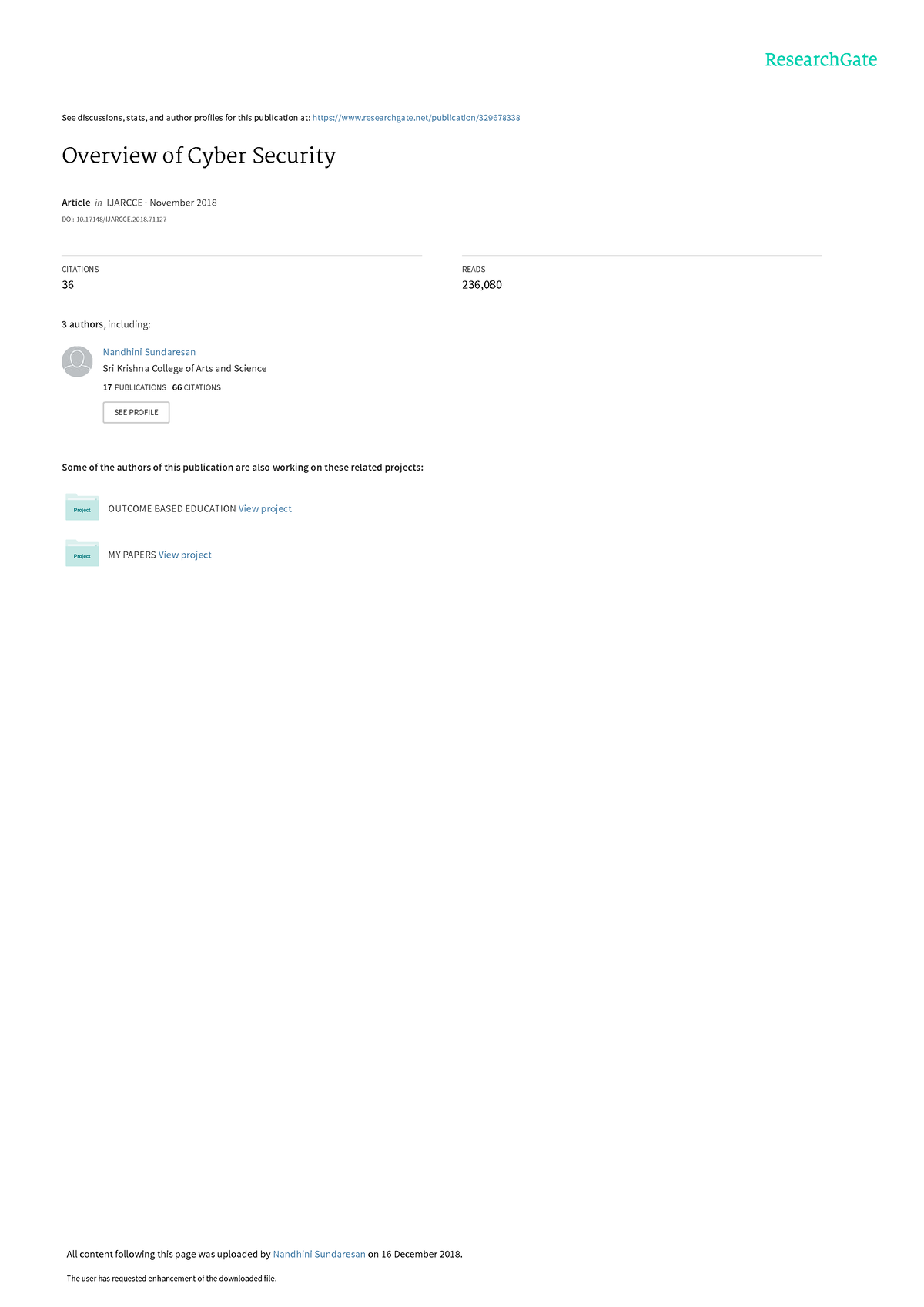The image is a small screenshot with a predominantly white background featuring primarily text-based content.

- **Top Right Corner:**
  - Blue serif text saying "Research Gate."

- **Below the Title:**
  - A very small line of text in black, followed by a blue URL.

- **Title:**
  - "Overview of Cybersecurity."

- **Main Body:**
  - A paragraph where the first word is in bold, but the rest of the text is too small to read.
  - A line of extremely small text follows.

- **Subsections:**
  - Two thin, dark gray vertical lines separate the content into two subsections.
    - **Left Subsection:**
      - Small, unreadable text followed by a bold number "36."
    - **Right Subsection:**
      - Small, unreadable text followed by a bold number "236,000."

- **Additional Details:**
  - Further down, another small line of text is present.
  - A dark gray circle with a white avatar icon is on the left, followed by blue text and black subtext.
  - Additional information follows below the subtext, including a small, unreadable button.

- **Bottom Sections:**
  - A bold line of text, followed by two rows of information each featuring a folder icon and black text.
  - A blue link labeled "View Project."

- **Footer:**
  - Two lines of black text, with the first line containing a blue link.

The overall structure indicates a professional document or online page detailing cybersecurity research, affiliated with Research Gate, including various user and project-related information.